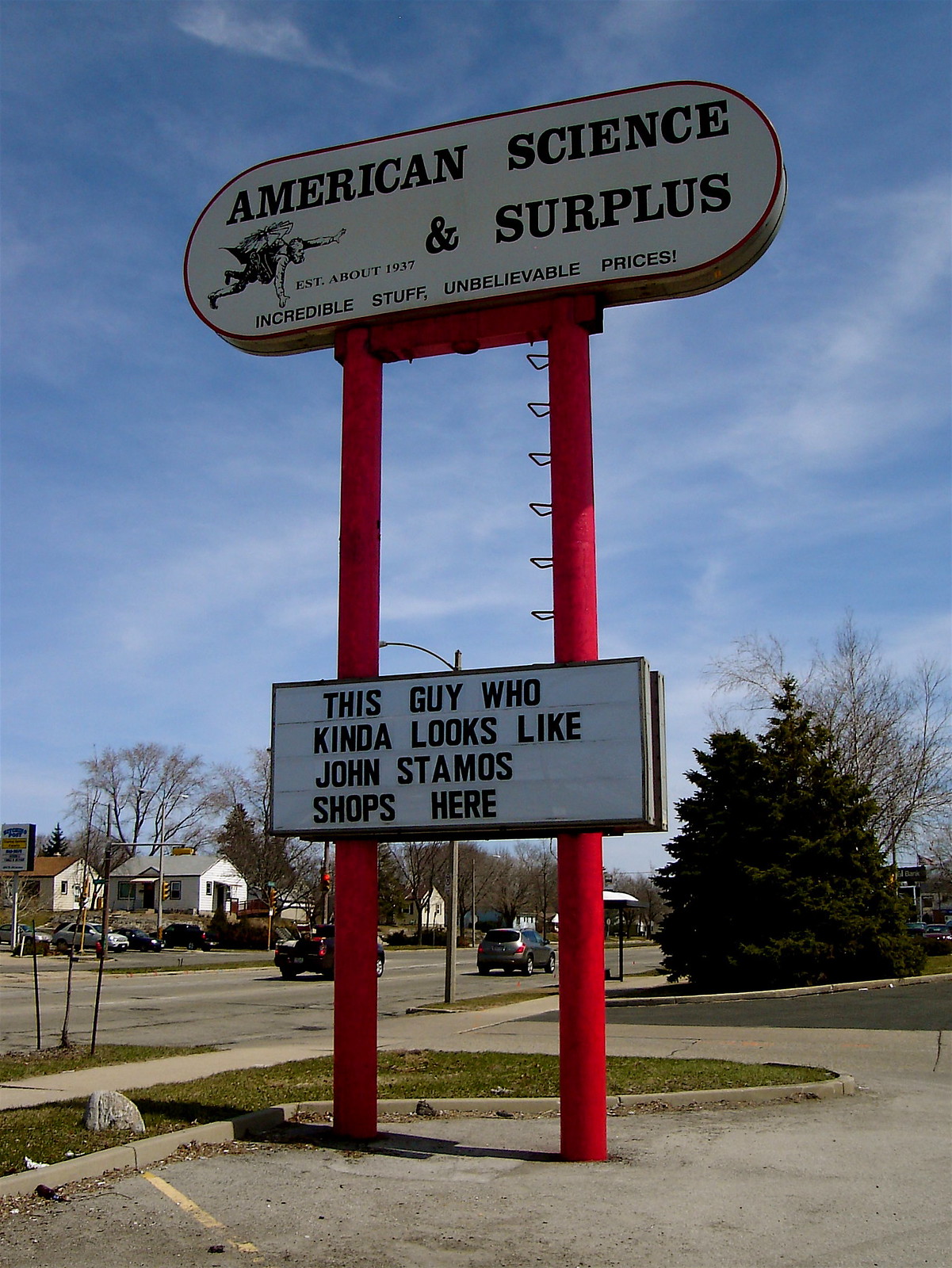A large, red street sign towers at the end of a parking lot, positioned near the intersection of what appears to be a four-way street. In the foreground, sidewalks and parking spaces lead up to the sign, which stands just before a yellow line marking. Clearly visible on the street is an SUV in motion and a truck carrying cargo in its bed. The sign prominently features the name "American Science and Surplus," accompanied by an illustration of a man hovering in mid-air. An inscription indicates that the store was established in 1937, boasting "incredible stuff, unbelievable prices." The sign's structure includes two long red supports extending downwards. There is also whimsical text suggesting that a man resembling John Stamos shops there, aimed at attracting more visitors. The background includes a scattering of trees, residential houses, and a clear blue sky, giving the scene a pleasant suburban feel.